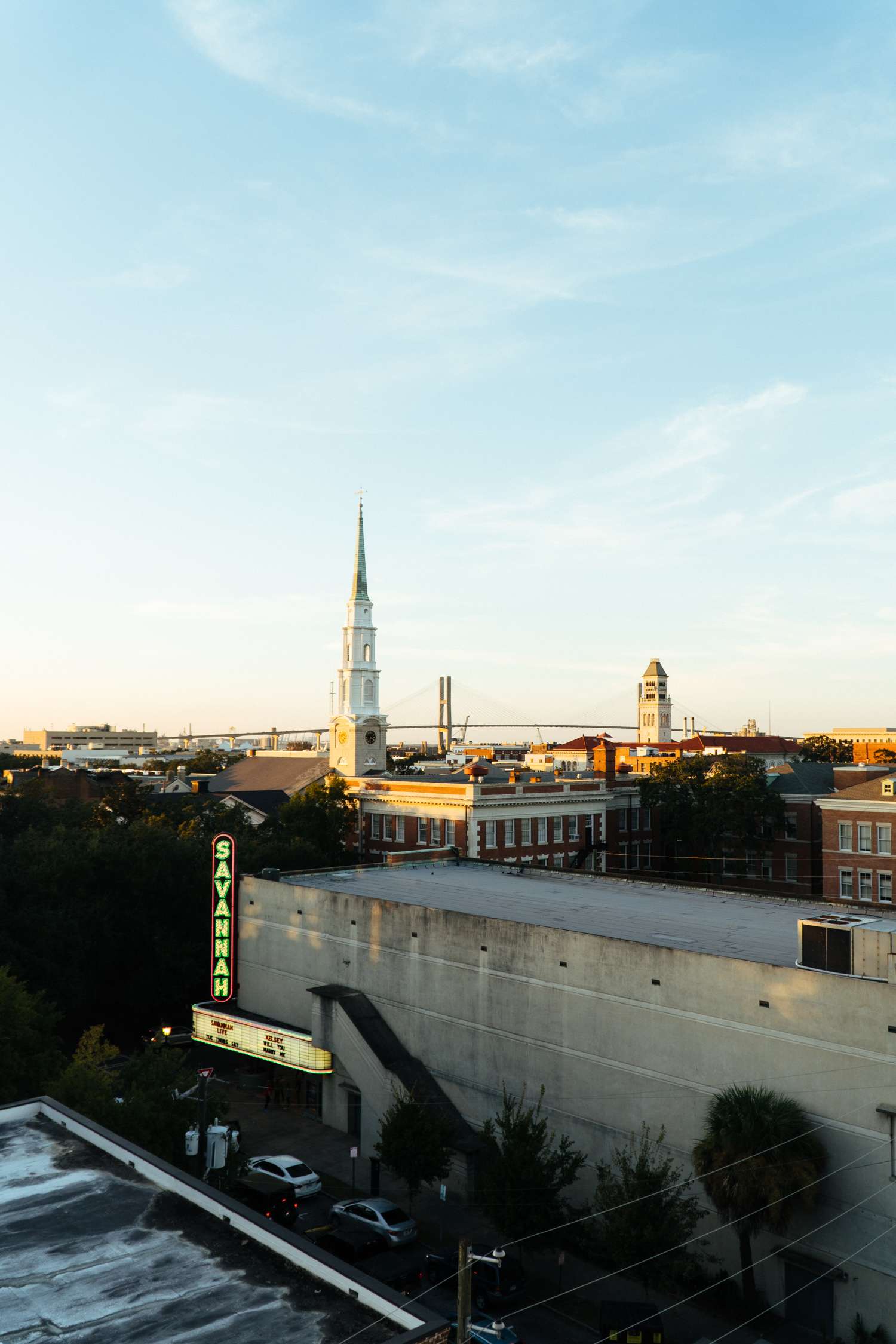The photograph captures a detailed cityscape of Savannah, taken from an elevated vantage point, likely a two to four-story building. The vertical portrait format emphasizes the layered depth of the scene. 

In the foreground, a long rectangular building dominates the view, featuring a striking vertical neon sign bearing the word "Savannah" in luminescent light green lettering on a black background with a red border. Below this sign, a marquee hints at the building possibly being a movie theater. Cars are parked in front of this structure, adding a dynamic urban touch.

The middle ground showcases the historic cityscape, with numerous red-brick federal-style buildings characterized by their box-like architecture and multiple windows. Notably, a tall, multi-leveled white church steeple rises above the surrounding structures, serving as a prominent landmark. Scattered throughout this scene are various trees of differing sizes, enhancing the sense of depth and greenery within the urban environment.

In the background, a distant span bridge stretches across the horizon, adding an element of connectivity to the composition. Power lines and poles are visible in the bottom right corner, reinforcing the urban setting.

The sky, which occupies the entire upper half of the photograph, is a serene light blue adorned with wispy, feather-like white clouds drifting gently across. The overall image combines architectural, natural, and infrastructural elements to provide a richly detailed depiction of Savannah's cityscape.